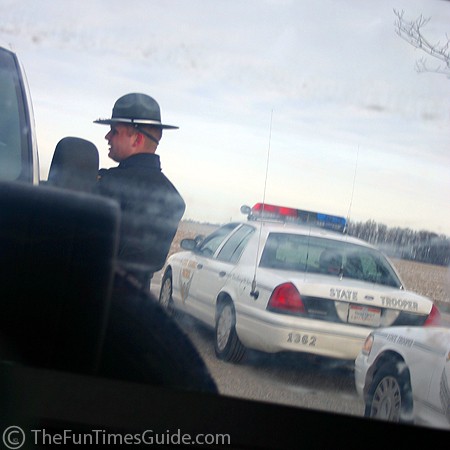The image depicts a state trooper, identifiable by his brimmed hat and dark uniform, standing on the left side of the frame. He appears to be in the process of speaking to someone through the passenger-side window of a vehicle, the right side of which and its side mirror are visible. The trooper's mouth is open as if he is conversing with the occupant. The scene also features the back half of his state trooper car, which is white with red and blue siren lights on top and the number 1362 marked on it. This car displays "state trooper" on its trunk. Positioned behind the trooper's car is another vehicle, likely a black sedan whose front end is not clearly discernible. In the background, one can observe tall, leafless trees amidst a partly cloudy sky with hues of white and gray. The entire scene unfolds on a road made of gray concrete, adjacent to a brownish field, suggesting a dull-colored day.